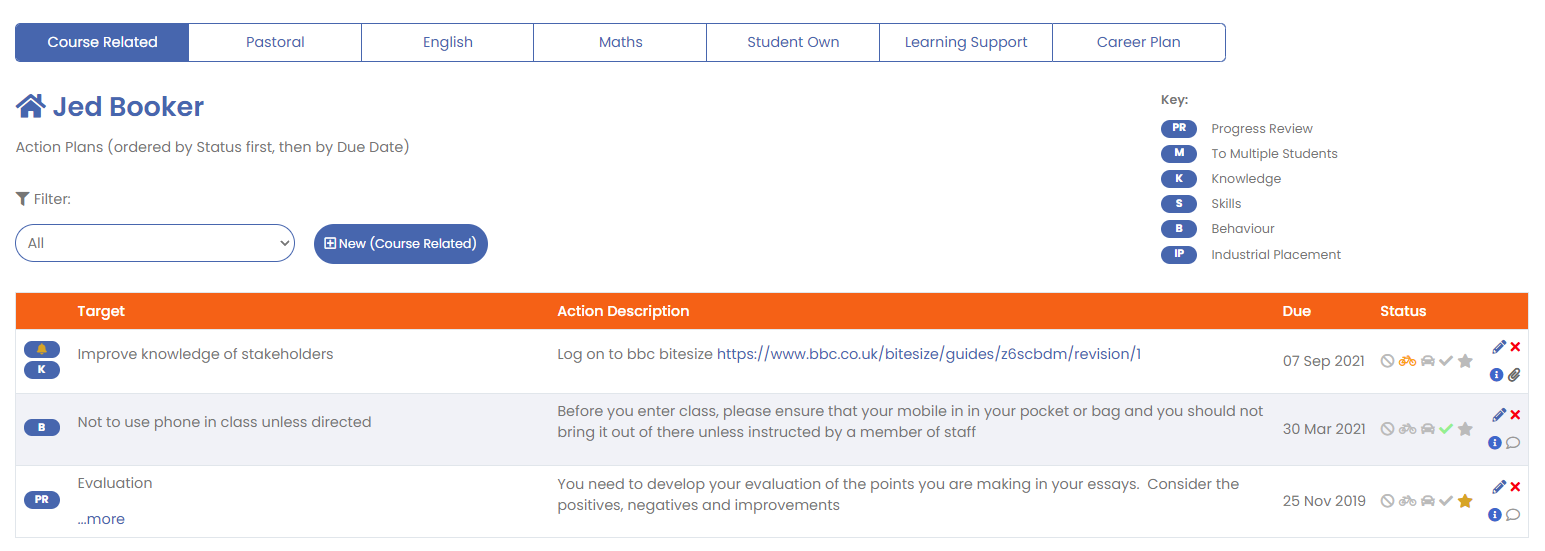The screenshot displays a computer interface tailored for someone named Jed Booker. Positioned in the upper left corner, the name "Jed Booker" appears next to a house icon. The screen is titled with "Action Plans Ordered by Status" followed by "then by Due Date." Below this title, there is an interactive box labeled "All" which users can click on, accompanied by a "New Course Related" option.

On the upper right side, a section labeled "Key" includes multiple blue ovals, each representing different categories: Progress Review, Multiple Students, Knowledge, Skills, Behavior, and Industrial Placement. Users can select different categories through these clickable options.

Dominating the middle of the interface, a prominent orange bar runs horizontally across the screen, containing white text headers: "Target," "Action Description," "Due," and "Status." Directly beneath these headers, the targets and actions are listed. One specific entry under "Target" reads: "Improve Knowledge of Stakeholders," with the corresponding "Action Description" instructing to "Log on to BBC Bitesize." The due date for this action is set to "7 September 2021," and the status is followed by a series of symbols, whose meanings are not immediately clear.